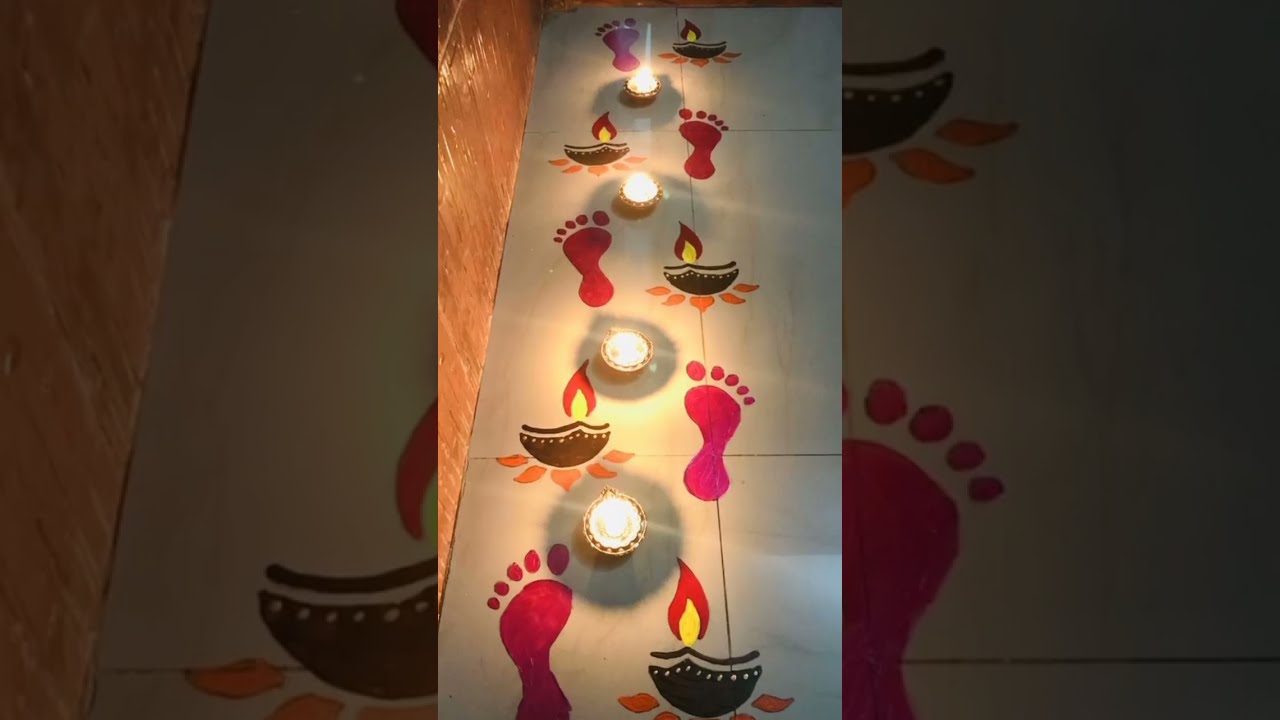The image depicts a detailed and artistic setup that appears to serve a meditative or perhaps religious purpose. In the center, there are four tea lights or small candles, each with a brown holder and a visible flame. Surrounding these lights are large, artistic footprints in shades of pink, cranberry, and light burgundy, alternating between left and right feet. These footprints are adorned with small, cartoonish symbols resembling flames or possibly Aladdin lamps, adding a Middle Eastern flair to the design. The entire scene, possibly laid out on the ground, is captured in a close-up photograph that appears to split the main image into three parts: the left and right sections show a slightly blurred, enlarged view of the central image, with the main colors being white, tan, and various shades of pink. The background includes a light orange or brown wall that is shiny and slightly faded. There are no people, animals, or vehicles in the image, suggesting an indoor setting, potentially a meditation area, religious space, or even an imaginative play area, although the presence of flames makes it less likely to be intended for children.